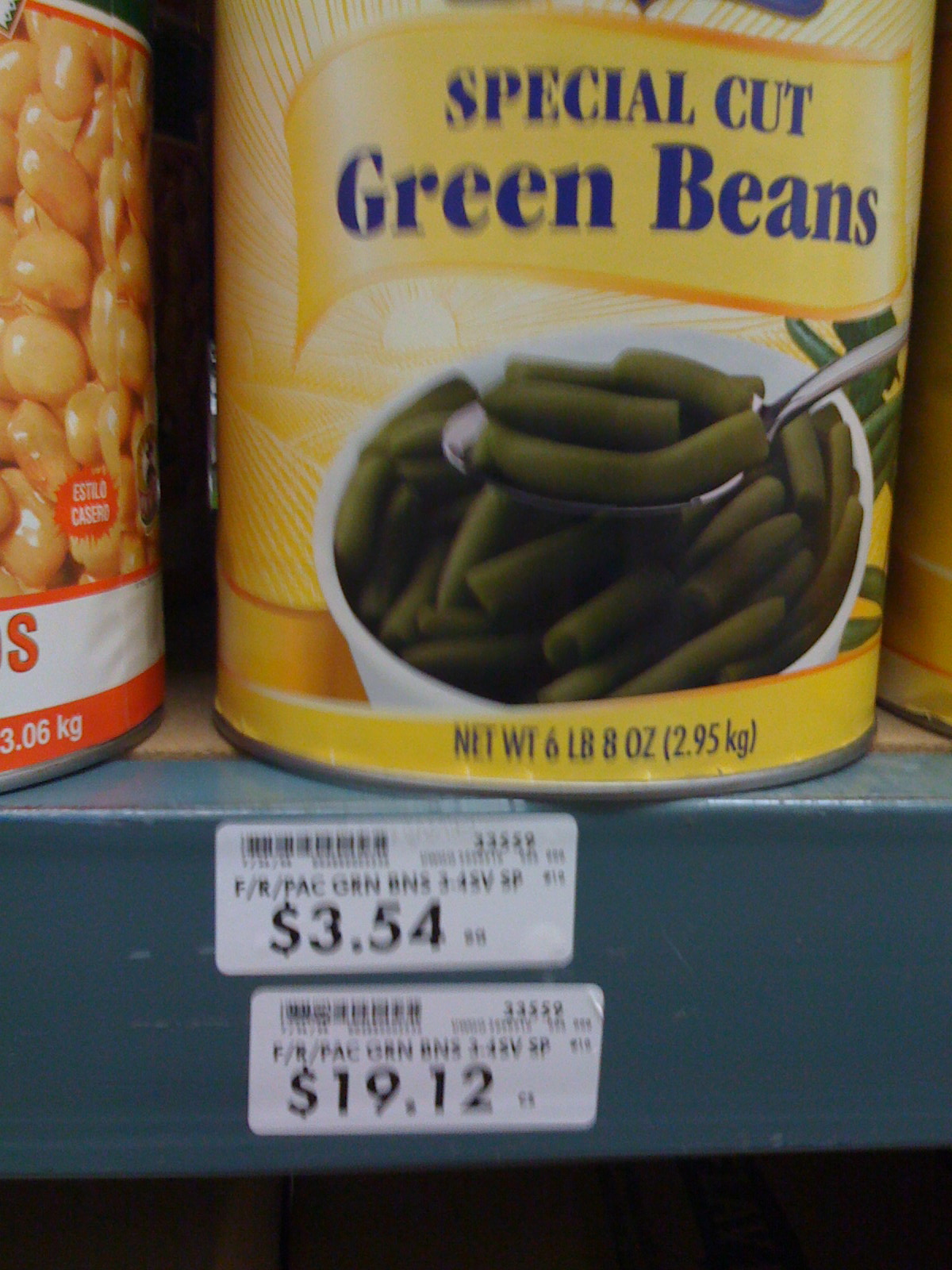The photograph depicts multiple cans of green beans displayed on a blue shelf in a grocery store. The focal point is a prominently positioned can with a predominantly yellow label, featuring an image of green beans in a white bowl. The label’s text is in blue and reads "Special Cut Green Beans," with additional information at the very bottom of the can that states "Net Weight 6 pounds 8 ounces (2.95 kilograms)." To the left of this main can, another can is partially visible, but its contents are indiscernible from the image. The shelf includes a price tag indicating a cost of $3.54, with a secondary tag beneath it displaying $19.12.